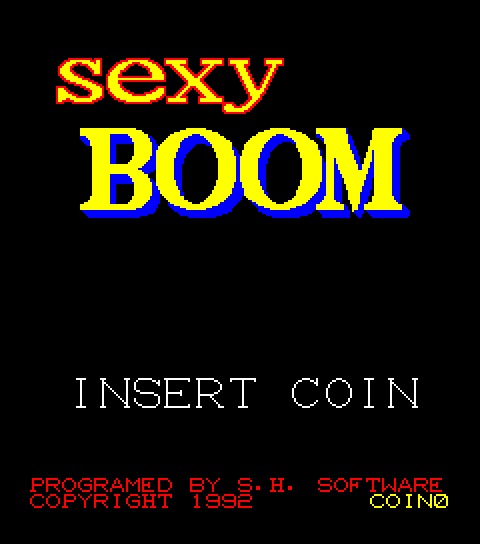This image resembles the opening screen of a vintage video game. The background is completely black, serving as a stark contrast to the vibrant text. At the top, the word "sexy" is prominently displayed in dark yellow letters with a red outline, rendered in a bold, video game style font. Directly beneath it, the word "boom" appears in light yellow letters with a distinct blue border. Following this, in white text, are the words "insert coin." Lower still, in red text, is the credit "programmed by S.H. Software," with "copyright 1992" marked just below it. Finally, in the bottom right corner, the yellow text reads "coin 0," completing the retro gaming aesthetic.